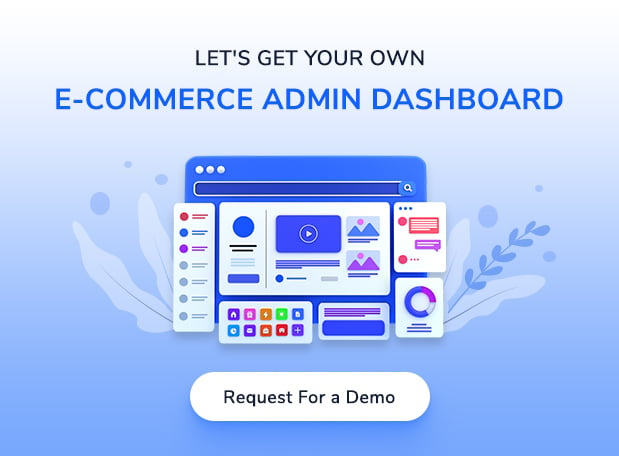This screenshot captures a demo page boasting a vibrant, light blue background adorned with subtle leaf graphics. Dominating the top section of the page is a bold, all-caps headline: "LET'S GET YOUR OWN" in black, followed by "ECOMMERCE ADMIN DASHBOARD" in blue. Beneath this text is a central graphic representing a browser window. The browser sports a blue background and an address bar, and it showcases a complex layout featuring six charts. Among these are a sidebar and two floating charts, while a large central chart occupies the majority of the space, indicative of an example template. Various example icons are displayed at the bottom of this browser graphic. Below, a prominent white button invites users to "REQUEST A DEMO." The background color transitions from light blue at the top to a darker shade as it descends, with additional leaf graphics accentuating the middle section behind the browser illustration.